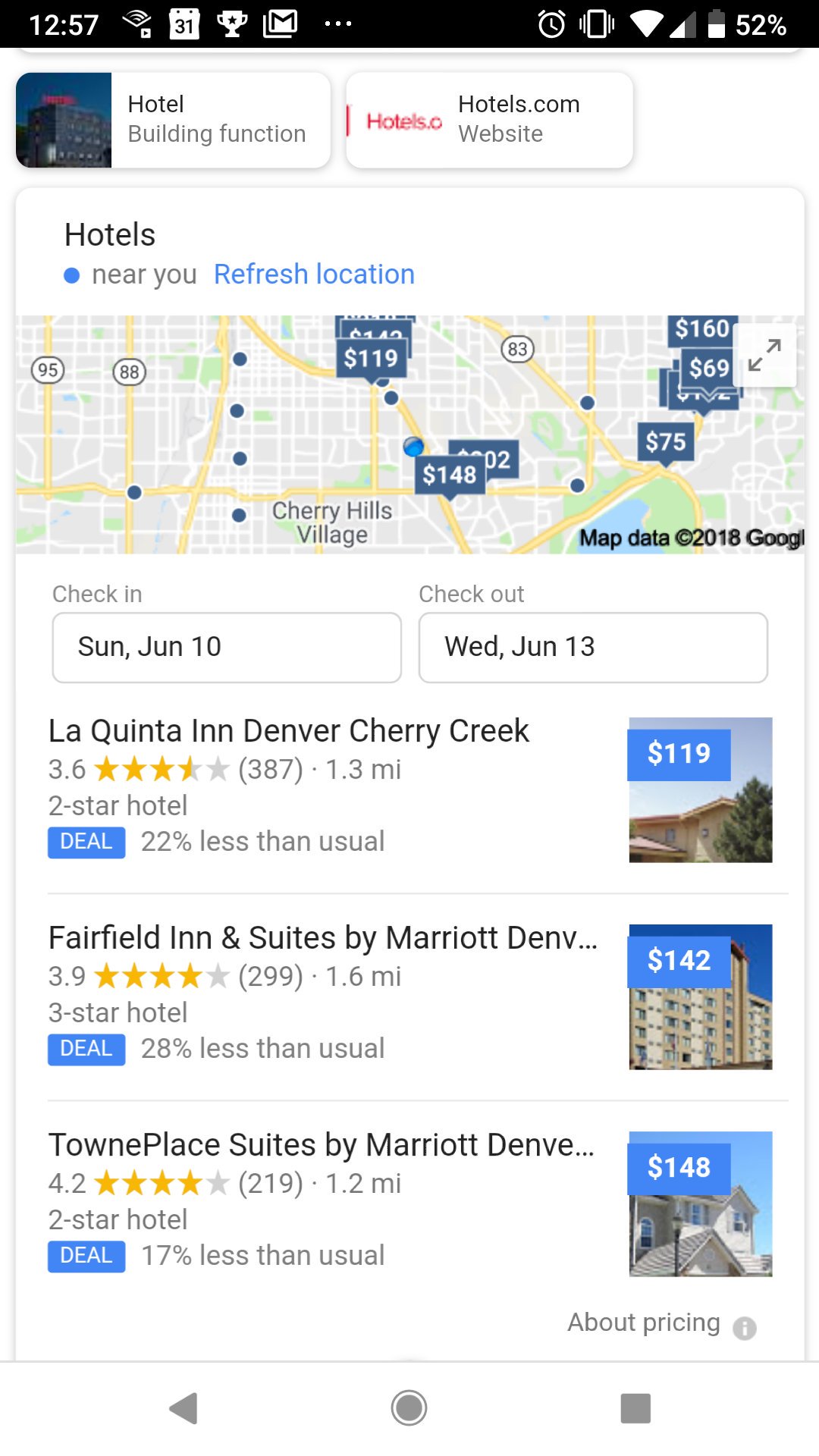The top-left corner of the screenshot shows the time as 12:57, along with a full Wi-Fi signal, half the cellular signal bar, and a battery at 52%. Adjacent to these, there are icons indicating a calendar, a trophy, and a horizontal ellipsis. Below these icons, two buttons are displayed: one labeled "Hotel building function" and another labeled "hotel.com website," followed by a caption "hotel near you."

A blue hyperlink reading "refresh location" precedes a Google Maps screenshot, showcasing various hotel prices in a specified area. Below the map, information about the check-in and check-out dates is provided, with text boxes displaying Sunday, June 10th for check-in and Wednesday, June 13th for check-out.

Further details include a highlighted hotel listing for La Quinta Inn, Denver, Cherry Creek. The listing notes the hotel has a rating of 3.6 stars from 387 ratings, is located 1.3 miles away, and is categorized as a two-star hotel. It also mentions a promotional discount of 22%, making the nightly rate $119, lower than the usual price.